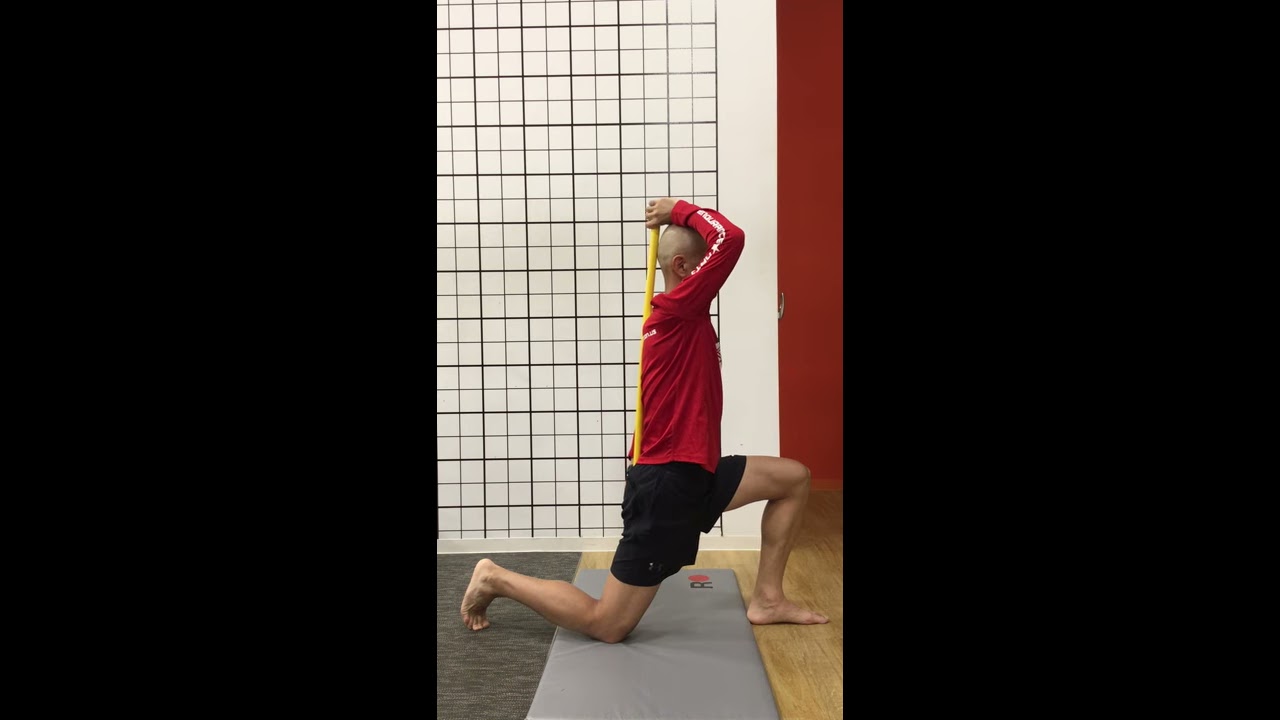The image captures a bald Caucasian man performing a kneeling lunge exercise on a gray rectangular mat, positioned centrally against a backdrop featuring a red wall and a cream-colored wall with a black geometrical pattern. He is wearing black shorts and a long red t-shirt adorned with white text on the right sleeve and back. His right knee is bent and touches the mat while his left foot extends beyond the mat onto the adjacent wooden parquet floor. The man holds a yellow stick in an overhead tricep press position, raising it behind his head and down his back, appearing to check his posture or back alignment. The setting includes dark carpet to the left of the mat and a wooden floor to the right, highlighting a contrast in floor textures. The thirds of the image to the left and right are pitch black, focusing the viewer’s attention on the central scene.